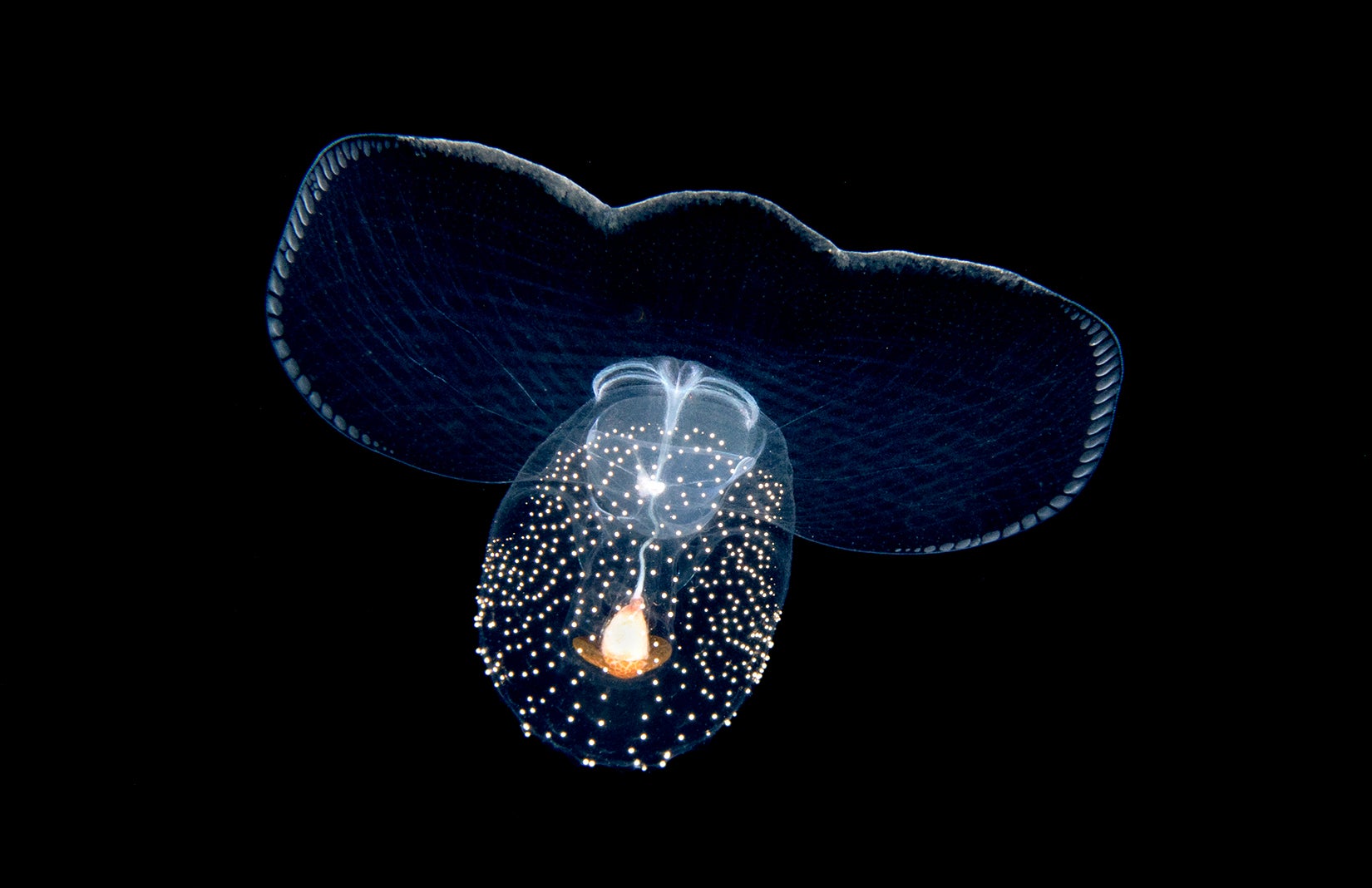The image vividly captures a marine organism, most likely a jellyfish, illuminated against a pitch-black background. At the center of the photograph is the jellyfish, glowing with luminous colors. Its jelly-like body showcases a bluish dome that resembles the shape of a stingray seen from above. Beneath the dome, fluorescent tentacles cascade down, highlighted by a warm orange glow at their core. Interspersed within these tentacles are numerous tiny white dots, resembling Christmas lights, adding to the ethereal quality of the creature. Central to the elegant structure is a larger light, drooping down like a glowing filament in a light bulb. The composition of the image, professional quality, and striking details suggest that it could feature in a National Geographic magazine or a marine biology documentary.